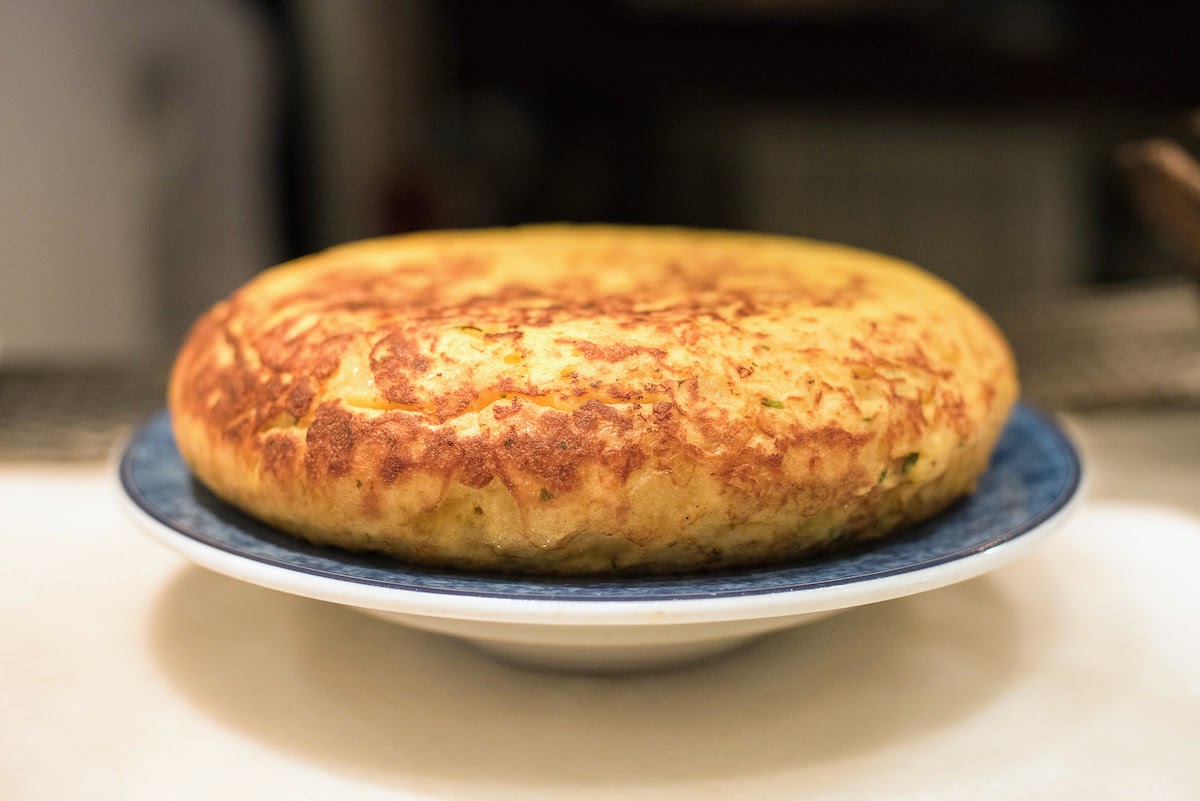This horizontally-aligned rectangular image showcases a close-up of a brown-crusted bagel resting on a white porcelain dish with a navy blue patterned rim. The bagel, which appears to have little green bits suggesting it's a jalapeno variety, displays a beautiful gradient of yellowish bread with browned edges. Positioned on a white table or counter, the dish casts a distinct shadow beneath it, hinting at overhead lighting. The shallow bowl in which the bagel sits contrasts its white exterior with a blue patterned interior. The background, though blurred, hints at a kitchen environment with darker colors and possibly a microwave on the left side, adding to the cozy, culinary setting.